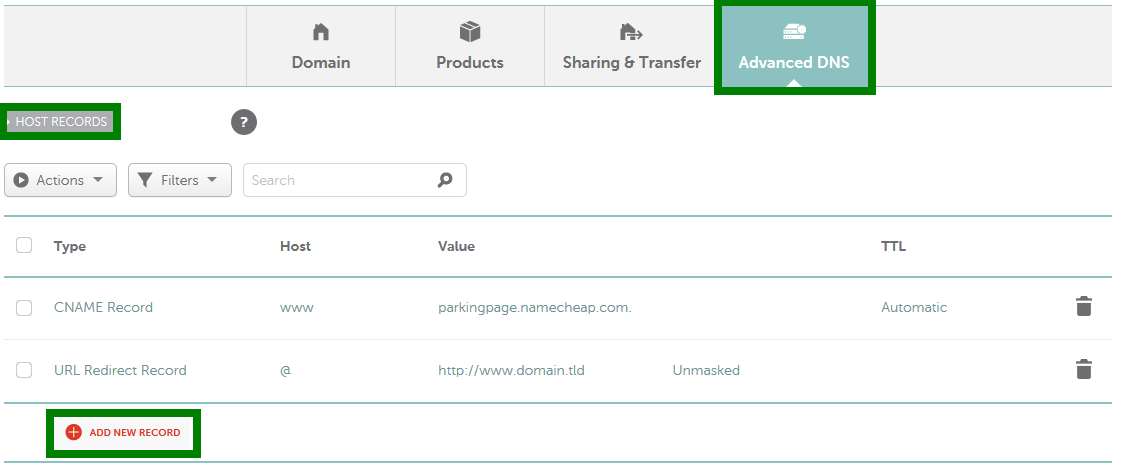This screenshot captures a detailed view of a database management interface on a computer's desktop or laptop. The software appears to focus on DNS (Domain Name System) management, featuring a clean white background complemented by black text and blue hyperlinks. At the top, a banner showcases navigation buttons labeled: "Domain," "Products," "Sharing and Transfer," and "Advanced DNS."

The "Host Records" and "Add New Records" buttons are prominently highlighted in green, each encased in green rectangles, indicating they are active or ready for interaction. Below the "Host Records" button, a drop-down labeled "Actions" is present, suggesting options for further actions related to host records. To the right, a "Filters" drop-down is positioned next to a search bar, facilitating efficient data filtering and retrieval.

The main content is structured in a table format, with column headers titled: "Type," "Host," "Value," and "TTL." Within the "Type" column, entries include "CNAME Record" and "URL Redirect Record." The "Host" column lists "www" and "@," while the "Value" column contains the entries "parkingpage.namecheap.com" and "http://www.domain.tld," explicitly marked as unmasked. The "TTL" column features "Automatic" and a blank entry. Each row is equipped with a trash icon at the far right, indicating the option to delete the corresponding record.

Additionally, a "Help" button is situated in the upper left corner, providing users with quick access to assistance resources. This comprehensive interface is designed for efficient navigation and management of DNS records, making it a robust tool for domain administration.